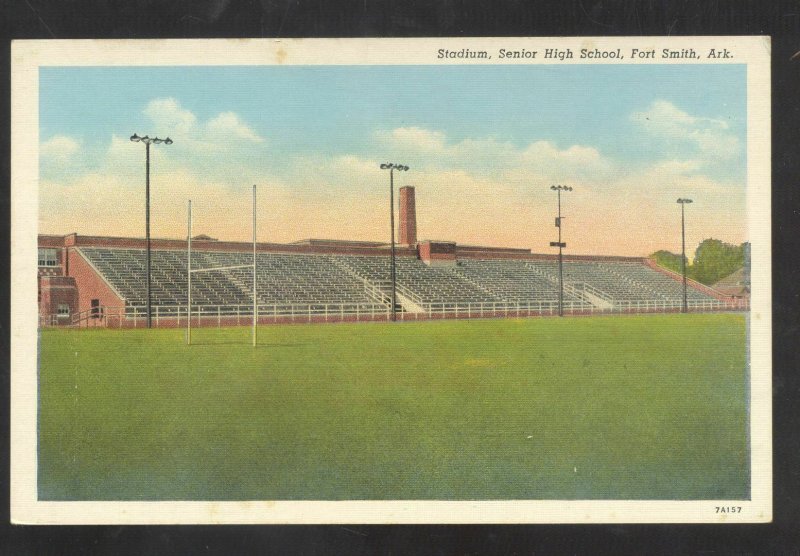The image appears to be a vintage postcard or illustration of a high school football stadium. The postcard is rectangular with a black border surrounding a white edge that frames the main image. The top right corner of the white border is printed with "Stadium, Senior High School, Fort Smith, Arkansas," and the bottom right corner displays the alphanumeric code "7A157."

The central image depicts an empty high school football stadium. The field is a lush green with white goalposts for American football, and a white fence separates the field from the stands. The stands themselves are constructed from red or brown brick, contrasting the black-and-white appearance of the bleachers. There are about 20 rows of seating divided into six large sections. Large field lights on wooden poles, each topped with clusters of four lights, flank the stadium, presumably for nighttime events. The sky is a hazy blend of blue and white, adding to the nostalgic feel of the image.